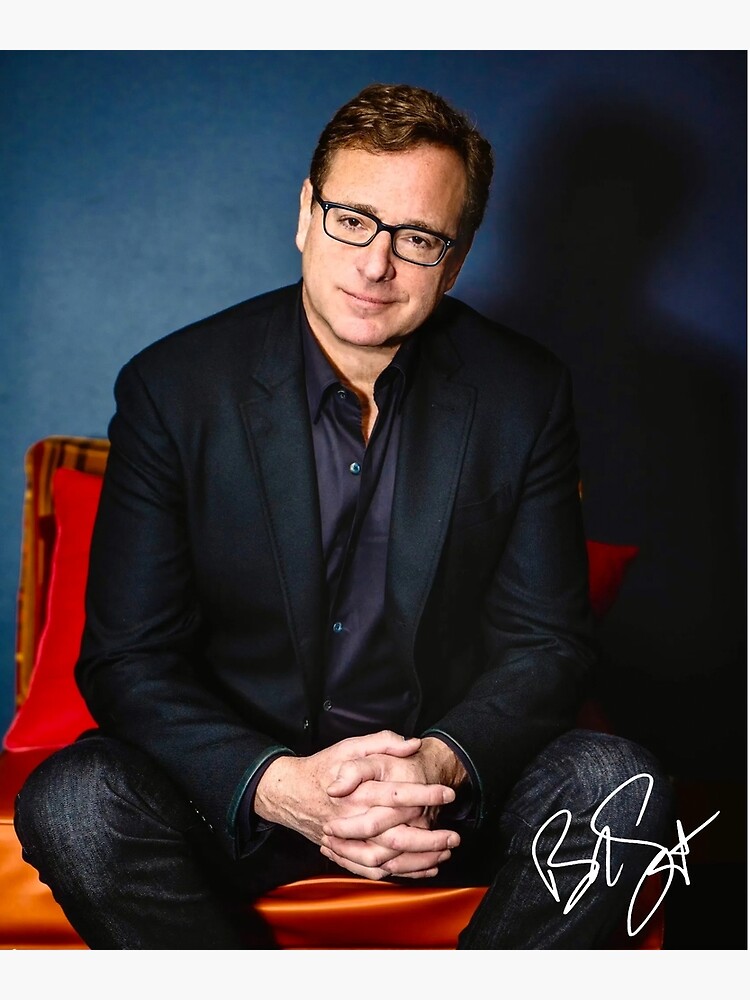The image is a vertical, autographed, color publicity photograph of the late comedian Bob Saget, best known for his role on Full House from the late '80s to early '90s. Bob is seated on the edge of an orange satin-upholstered sofa or chair, with a red throw pillow behind him. He is dressed in black jeans, a black blazer, and a dark gray button-down shirt. His hands are clasped in a relaxed manner between his knees, and he is smiling gently with his head slightly cocked to the side. Bob is wearing glasses with black frames, and his hair is neatly combed. The background features a blue wall with a shadow cast upon it. His autograph is prominently displayed in white marker at the bottom right corner of the photograph.